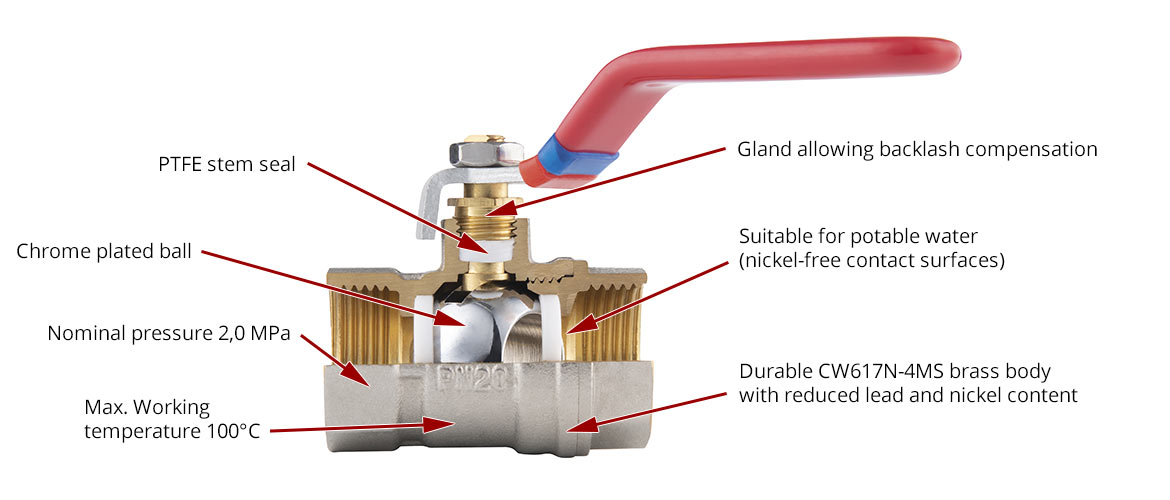This detailed image is a digitally created cutaway diagram of a mechanical valve with a red handle. The valve features a steel base, exposing its internal components through the cutaway. At the top of the valve, an arrow indicates the "gland allowing backlash compensation." Below this is a "PTFE stem seal" followed by a "chrome-plated ball" inside the structure. The valve also includes "nickel-free contact surfaces suitable for potable water." Additional specifications provided are a nominal pressure of 2.0 MPa and a maximum working temperature of 100 degrees Celsius. The body of the valve is constructed from durable CW617N-4MS brass with reduced lead and nickel content. The red handle is angled at about 45 degrees, designed for operation, and made of rubber for ease of use. Overall, the diagram meticulously labels and highlights the various parts and noteworthy features of the valve.